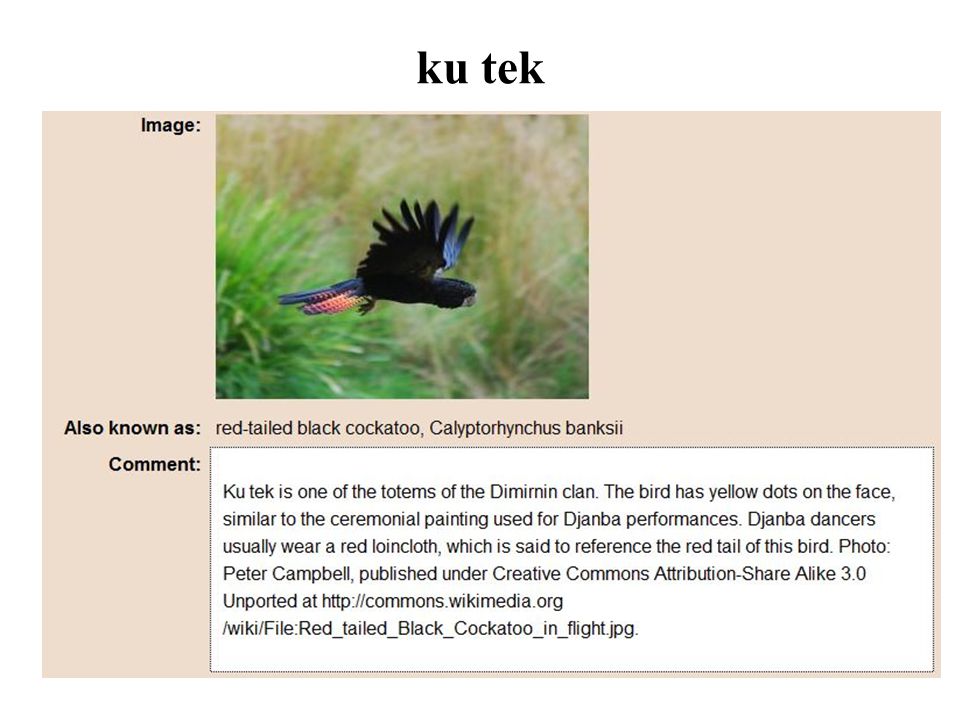The image depicts a black cockatoo, specifically the red-tailed black cockatoo (Calliptorhynchus banksii), in mid-flight against an outdoor nature backdrop. The cockatoo is characterized by its black plumage, vibrant red tail, spiky wings, and distinct yellow dots on its face that resemble ceremonial paintings. The picture is laid out like a book page—possibly for a nature or ornithology book—with "KUTEK" (K-U-T-E-K) written at the top in black text. Below the bird image, there's an extensive descriptive caption with both common and scientific names, associating the bird as a totem of the Dimirnin clan. It highlights cultural connections, noting that janba dancers mimic the bird's yellow facial dots and red tail with their ceremonial attire. A credit mentions the photo is by Peter Campbell, published under Creative Commons Attribution ShareAlike 3.0 Unported at Wikimedia. The bottom part of the image includes a box for comments. The overall palette includes colors such as blue, black, orange, purple, green, beige, white, and brown, adding depth to the bird’s vivid portrayal.